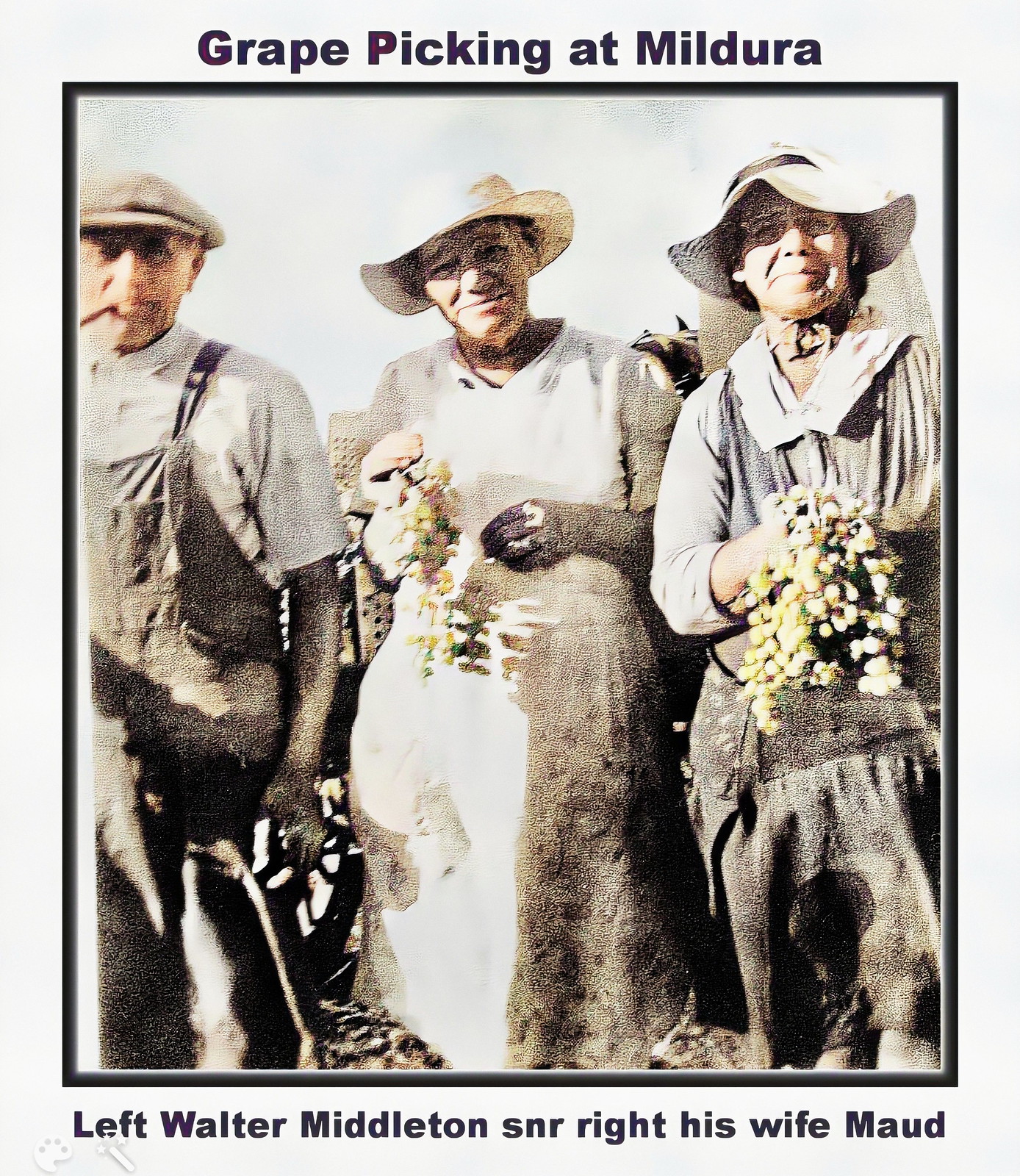In this detailed, vintage-style color image with a gray border, titled "Grape Picking at Mildura" in purple text at the top, Walter Middleton Sr. stands on the left, wearing a hat, overalls, and a shirt. To his right is his wife, Maud, who is on the far right of the image, dressed in a blue-colored dress and wearing glasses. Positioned between Walter and Maud is another woman in a white dress holding a bunch of grapes. The three individuals are outdoors, likely in the middle of the day, with a backdrop suggesting an agricultural setting. The image, featuring colors such as off-white, black, gray, tan, yellow, green, and various shades of gray, has a nostalgic feel reminiscent of the 1950s or 60s. The text at the bottom reiterates the identities of the figures: "Left, Walter Middleton Sr. Right, his wife Maud."